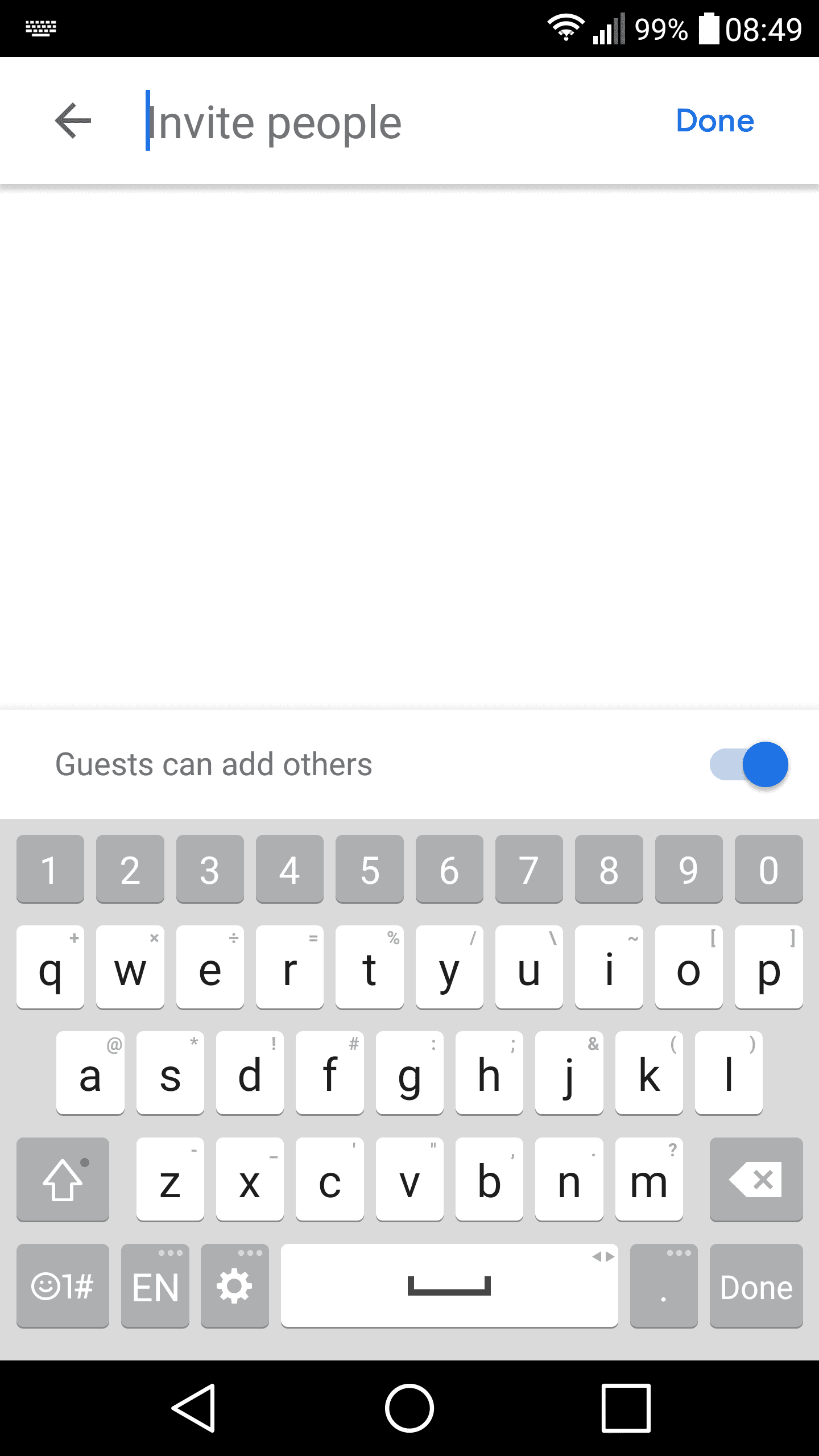This image appears to be a screenshot taken on a cell phone, featuring a user interface likely related to a communication or event-invitation app. The layout consists of a predominantly white background bordered by black rectangles at the top and bottom.

**Top Section:**  
The black rectangle at the top displays several icons on the right side, along with the current time, “8:49.” 

**Main Interface:**  
Directly below this, in a white input field marked by a blinking cursor, it says "Invite people.” To the left of this input field is an arrow pointing left, and to the right, the word “Done” appears in blue text, indicating a clickable button.

**Middle Section:**  
Beneath the input field and a segment of empty white space, a gray line separates another instruction: “Guests can add others.” To the immediate right, there is a blue toggle switch, which is turned on, signifying that guests have permission to add other invitees.

**Keyboard Interface:**  
Occupying the lower portion of the screen is the on-screen keyboard. The keyboard’s number keys and special characters are set against a slightly darker gray background with white lettering, whereas the alphabetical keys have a white background with black lettering. The space bar at the bottom of the keyboard follows this same white background with black text.

**Bottom Section:**  
At the very bottom of the screen, another black rectangle houses three navigation buttons: a triangle pointing left on the left side, a circle in the center, and a square on the right side. These are standard navigation icons in many mobile operating systems.

The image does not display the entire screen’s edge, focusing instead on this central interface.